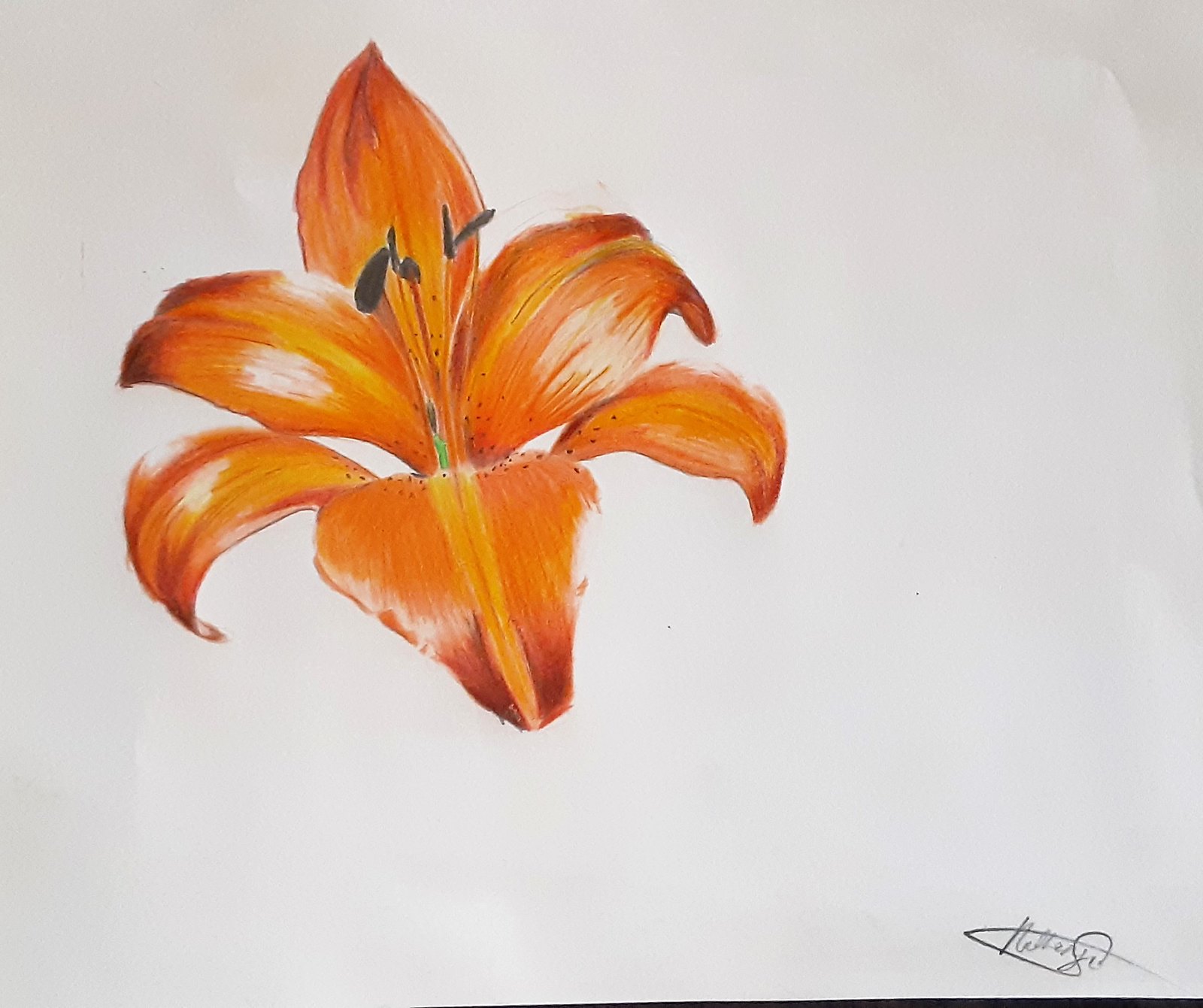This is a detailed photograph of a hand-drawn or painted image of a vibrant orange flower, likely a tiger lily, on a piece of white printer paper. The flower, situated in the upper left corner, has six boldly colored petals each featuring a yellow stripe down the center. In the middle of the bloom, there are three slender, stick-like protrusions with black dots atop them, presumably representing seeds or stamens. The paper shows visible wrinkles, particularly in the upper right and lower left corners. The bloom is depicted alone without a stem or any other parts of the plant. The bottom right corner of the paper reveals a barely legible signature, possibly saying "Kelly," hinting at the artist's name.